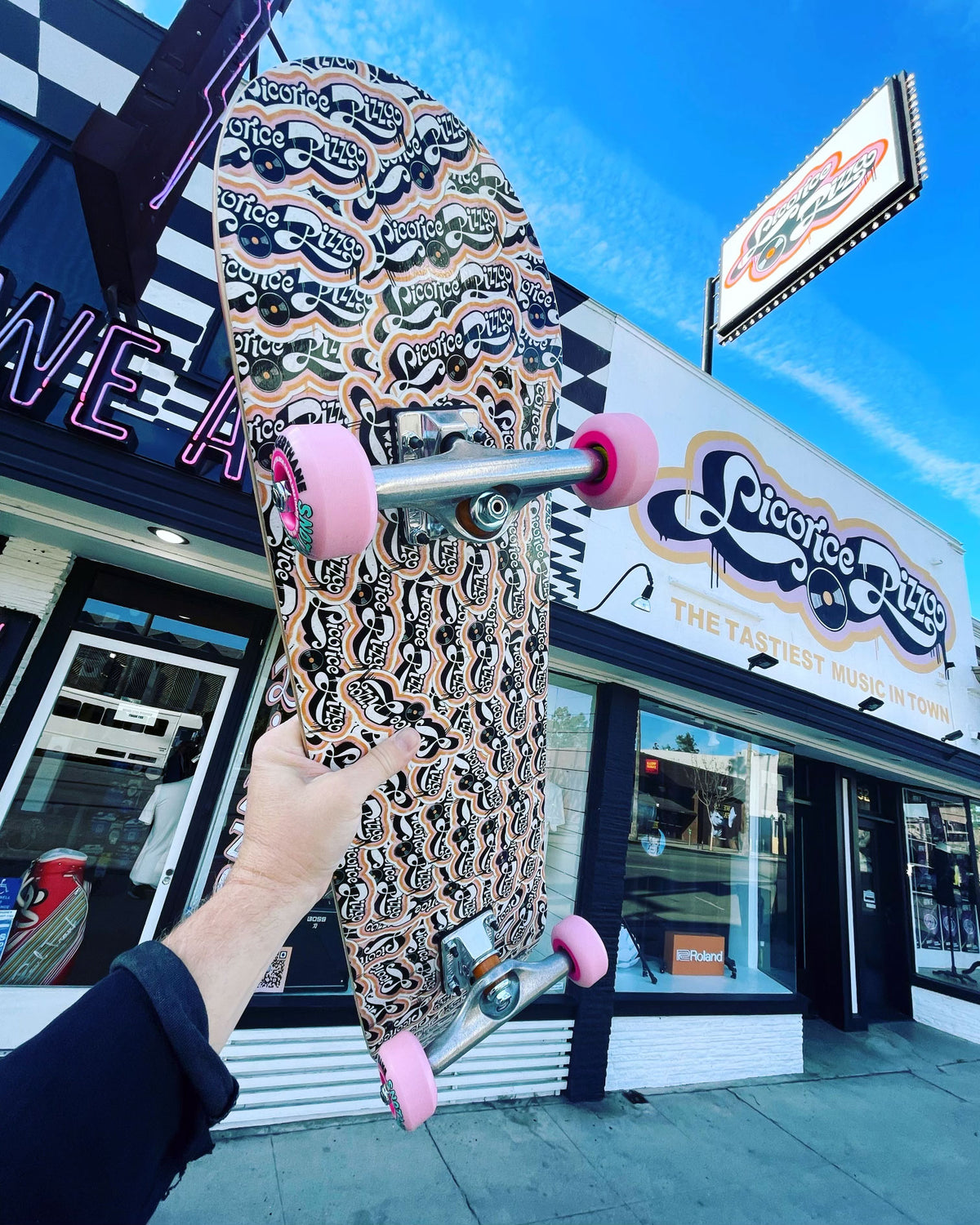In front of a white building accented with black trim, a person in a three-quarter-length blue top and black sleeve holds up a skateboard, displaying its underside prominently. The skateboard, which features pink wheels and a silver axle, is covered with the repeated logo "Licorice Pizzey" in black and white against a pink base. The storefront behind, named "Licorice Pizzey: The Tastiest Music in Town," has matching signage with a graffiti-style logo and large windows. The scene is framed by a clear blue sky with a hint of a white trail, possibly from a passing airplane, adding a dynamic backdrop to this unique urban tableau.